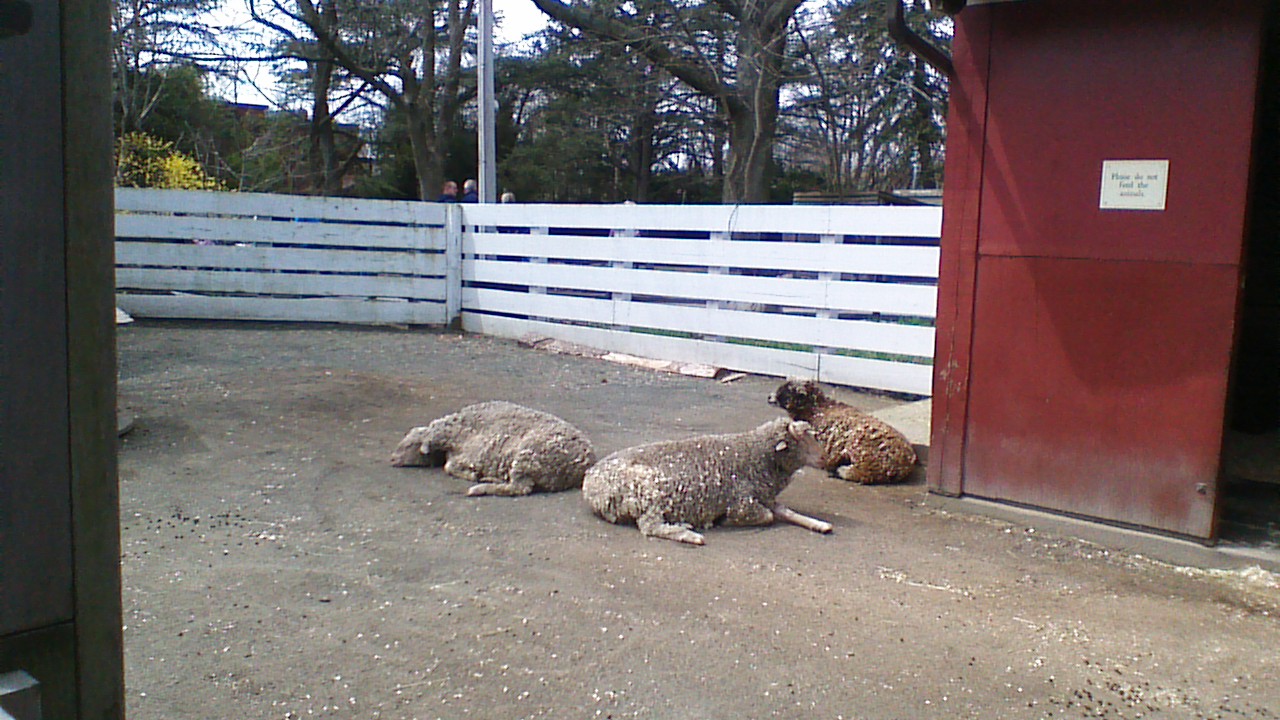In this photograph, the viewer is looking out from a red barn door that opens inward to reveal a dirt and gravel walkway. A white sign on the barn door reads, "Please don't feed the animals." Just beyond the doorway, three sheep are lying on the ground. Two sheep have dirty, grayish wool, while the third sheep has brown wool with a black face. A tall, white wooden fence with horizontal slats encircles the area, separating the animals from the outside world where a few people can be seen walking by. Behind the fence, tall green trees and some shrubs contribute to the foliage-rich background. To the right of the image, part of another building is faintly visible, while towards the left, there appears to be the rusted lower section of the shed. The overall scene suggests a tranquil, rustic enclosure possibly part of a zoo or farm.